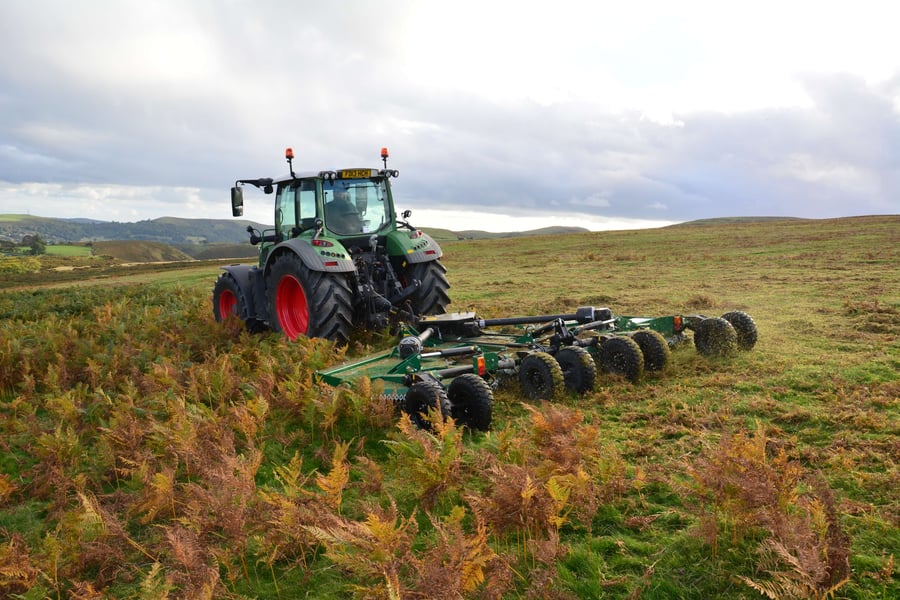The image portrays a green tractor with a mowing device on a large, open farmland. The tractor's two large front wheels with red rims are complemented by smaller wheels on the back. The mowing device in the front has a flat structure with multiple sets of wheels. There's a figure visible through the clear glass windshield, operating the vehicle, but their details aren't discernible. The scene shows a contrast between the brown, yellow, and green wheat on the left and the freshly mowed, light green and brown grass around and ahead of the tractor. Bushy reddish and orange plants occupy the bottom left corner. The background features rolling hills and a cloudy sky, enhancing the vastness of the landscape.